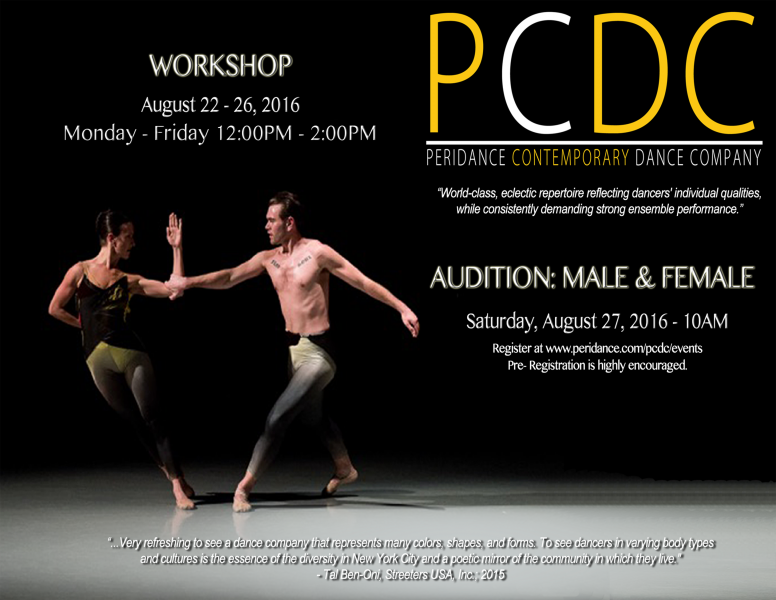The image features a striking advertisement set against a black background with a white stage at the bottom. On the left, a dynamic photograph captures a duo of dancers: a woman on the left in a full-body leotard with her arm raised in an L shape, and a man to her right, shirtless and wearing tights, gripping her arm. Above them, in white lettering, it reads, "Workshop August 22nd to 26th, 2016, Monday to Friday, 12 p.m. to 2 p.m." Prominently displayed in the top right corner are the letters "PCDC," with the first C in white and the rest in yellow. Below this, the text "Perry Dance Contemporary Dance Company" appears, with "Contemporary" uniquely highlighted in yellow. A quote beneath touts, "World-class eclectic repertoire reflecting dancers' individual qualities while consistently demanding strong ensemble performance." Further down, the ad announces an "Audition Male and Female Saturday, August 27th, 2016, 10 a.m." Additional details, including a web URL for registration, are provided at the bottom.